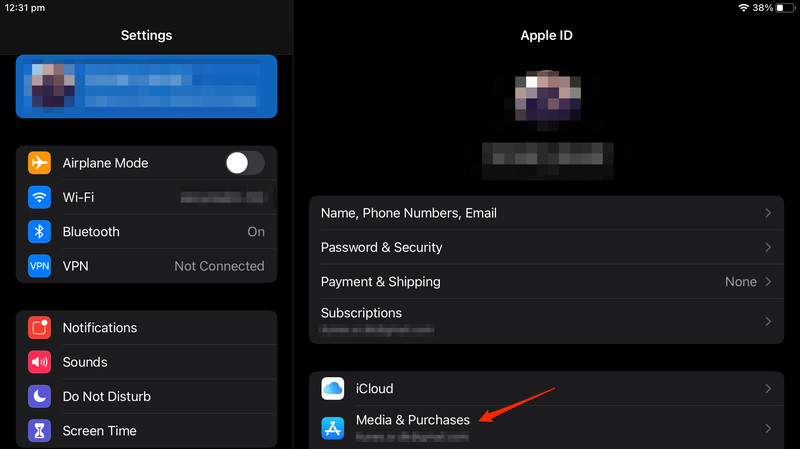This image, displayed in landscape orientation, captures a segment of a cell phone screen with a black background. At the top left corner, white text indicates the time as "12:31 PM." Adjacent to the time display, icons reveal the phone's signal strength, a "38%" battery level, and a lateral battery icon.

The screen showcases a settings menu split into two vertical panels. On the left, there's a section titled "Settings" in white text. Below, various settings categories are listed: Airplane Mode (selected), Wi-Fi, Bluetooth, VPN, Notifications, Sounds, Do Not Disturb, and Screen Time.

The right vertical panel occupies approximately two-thirds of the screen. At the top, it features the title "Apple ID" alongside a blurred-out icon and identification image. Following this are several options in white lettering: "Name, Phone Numbers, Email," "Password & Security," "Payment & Shipping," and "Subscription." Further down, there are selections for "iCloud" and "Media & Purchases." A prominent red arrow is drawn pointing to "Media & Purchases," starting from the top right of the option word and ending just to the right of it.